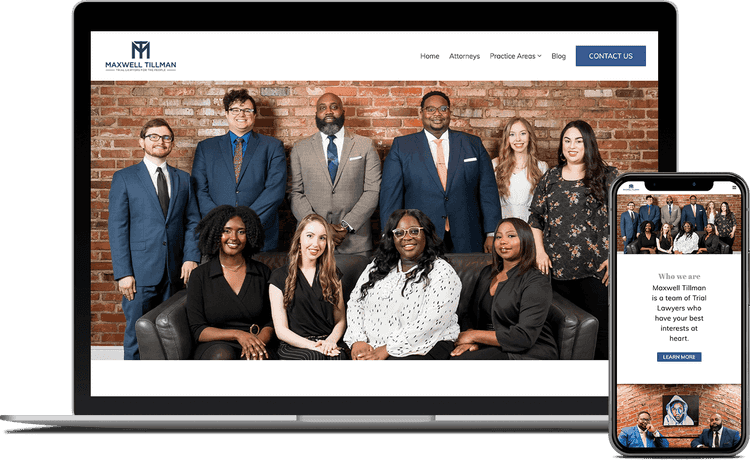In this detailed image, a computer or laptop and a mobile device are prominently featured. On the screen, there is a website displaying a snapshot of 10 individuals, consisting of 4 males and 6 females. The males are dressed in suits, with 3 out of the 4 wearing glasses. Among the females, one is also wearing glasses. The group includes a mix of ethnicities: 3 Caucasian males, 2 Black males, 3 Caucasian females, and 2 Black females.

In the top left corner of the screen, the name "Maxwell Tillman" is displayed, indicating the identity of the team. Positioned at the top right of the screen are several navigation options: "Home," "Attorneys," "Practice Areas," "Blog," "Contact Us," and "Who We Are." Below these options, there is a highlighted statement which reads, "Maxwell Tillman is a team of trial lawyers who have your best interest at heart. Learn more," suggesting a focus on client advocacy and professional legal services.